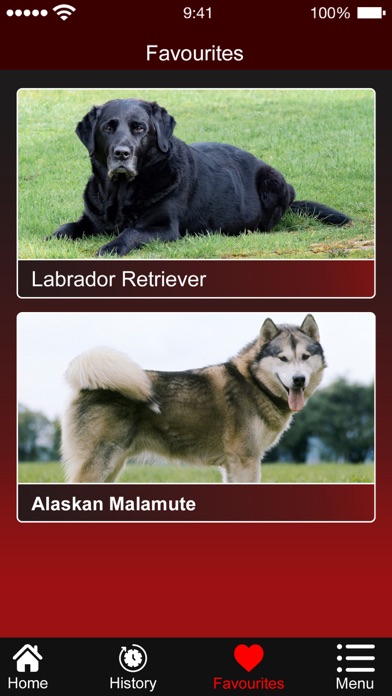The image is a detailed screenshot taken from a phone, showcasing a user interface against a gradient red background that transitions from lighter red at the bottom to black at the top. At the very top of the screenshot, the status bar indicates a full signal strength, the time displayed as 9:41 (with no AM or PM distinction), and a battery icon showing 100% charge.

Below the status bar, on a dark maroon header, the word "Favourites" is prominently displayed, spelled in British English. The first photograph features a black Labrador Retriever lying down on green grass with a caption in white text reading "Labrador Retriever." This photograph is set against the darker section of the gradient background.

Directly beneath the Labrador Retriever, another photograph captures an Alaskan Malamute standing outdoors, with a blue sky, trees, and grass visible in the background. The dog has gray and tan fur, a white face, and pointed ears, with its mouth partially open and its pink tongue visible. This image is also captioned in white text, "Alaskan Malamute," set within the dark maroon section of the background, consistent with the first photograph's layout.

At the bottom of the screen, icons are neatly arranged on a black bar, each accompanied by white labels. From left to right, there is a home icon labeled "Home," a clock icon labeled "History," a red heart icon labeled "Favourites," and three horizontal lines with bullet points labeled "Menu."

This composition effectively highlights the two favorite dogs of the user, displayed with cohesive text and detailed images, all framed within a thoughtfully designed gradient background on the phone screen.